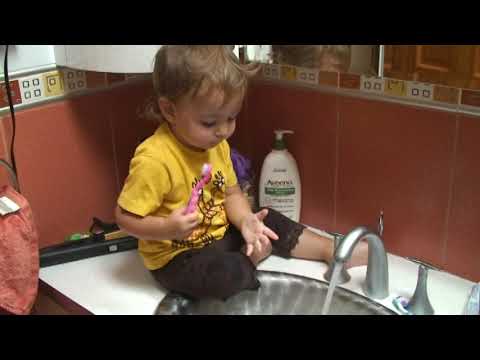A detailed photograph shows a young child, approximately two years old, sitting cross-legged on a white bathroom countertop next to a silver sink with a stainless steel faucet, from which water is visibly running. The child, of Caucasian descent, is wearing a yellow T-shirt adorned with black writing and black leggings featuring ruffled bottoms. In the child's right hand, they hold a pink toothbrush with a white bristle tip, held upright, while the left hand is outstretched with fingers spread, as though reacting to the water from the faucet. 

The bathroom wall behind the child features off-red tiling with a distinctive pattern consisting of squares in white, yellow, and darker shades of red. Other notable items include an Aveeno lotion bottle with green markings situated to the right of the child and a flat iron positioned nearby. Additionally, a pink-coral hand towel hangs on a towel ring in the background, and the top right corner of the image reveals a portion of a mirror reflecting the child's head and a brown wooden door.